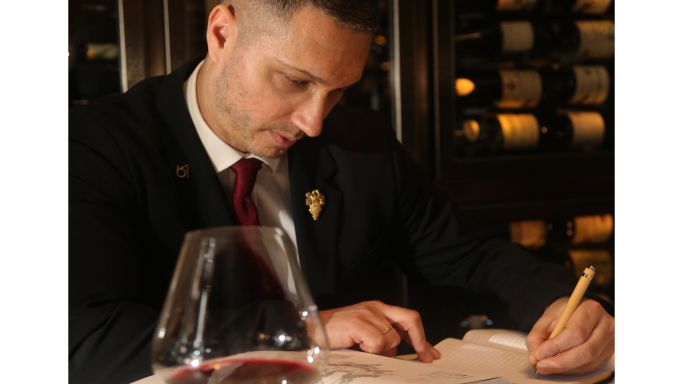The color photograph captures a man in a dark suit jacket, accented with a gold pin on the lapel, a white collared shirt, and a red tie. He is seated at a table, deeply focused on writing or drawing in an open book with white pages. His left hand holds a yellow pen, while his right hand steadies the book, revealing a gold wedding band. The man, who sports a light beard and short hair shaved on the sides, appears meticulous in his task. In the foreground, a glass of red wine adds a touch of elegance. Behind him, the dimly lit background features several wine bottles arranged horizontally within a dark brown wooden wine case, protected by glass doors. The white labels on the bottles stand out, suggesting the setting might be a sophisticated wine cellar.